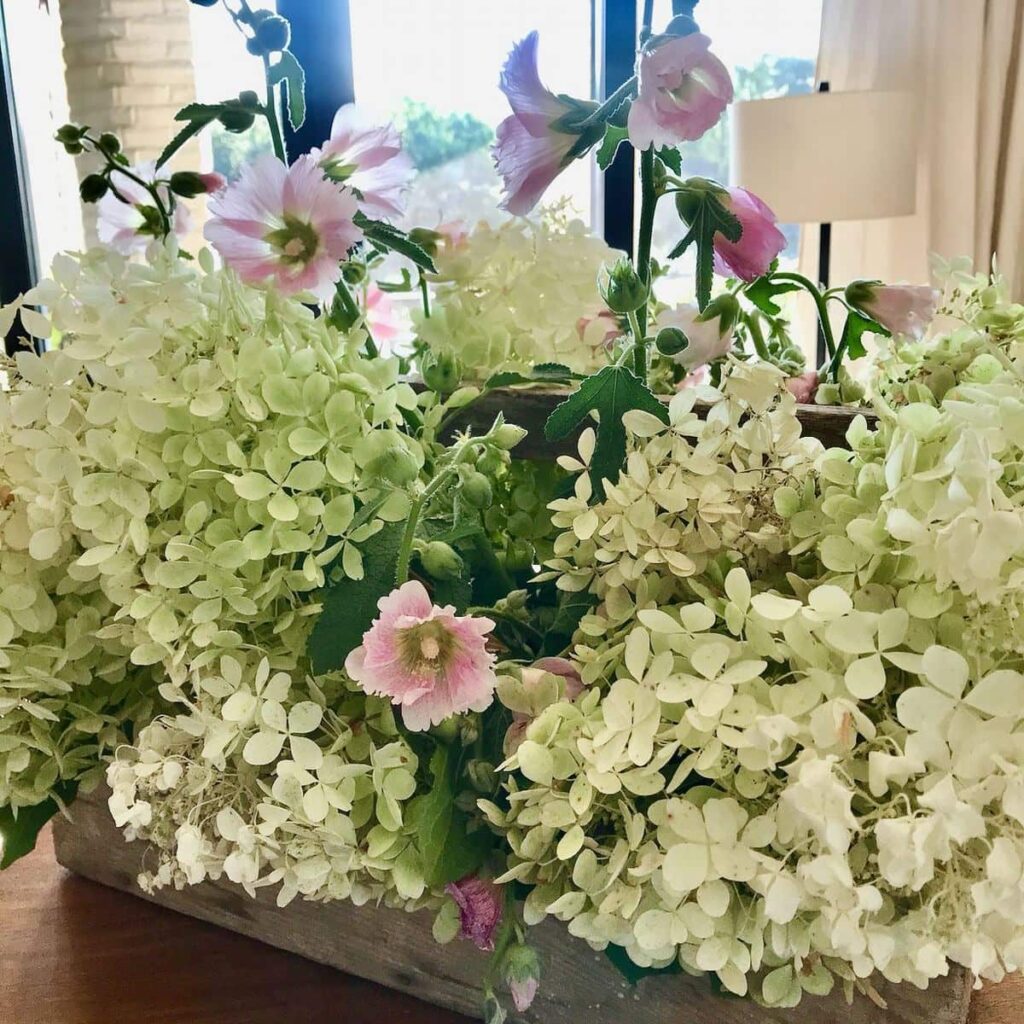The image showcases a lush flower arrangement meticulously placed in a wooden box, perched on a wooden hutch in front of a lamp by a window. Dominating the bouquet are beautiful white hydrangeas and fully-opened pink peonies, with potential additions of white almond-shaped flowers and greenery hinting at snapdragons or the Rose of Sharon. The flowers, freshly cut from bushes, spill elegantly over the edges of the box, creating a predominantly white and light green palette with subtle pink accents. In the background, white blinds and a white lampshade on the wooden hutch blend harmoniously with the surrounding decor, which includes white brick seen through the window and white sheer curtains, all bathed in natural sunlight streaming in.